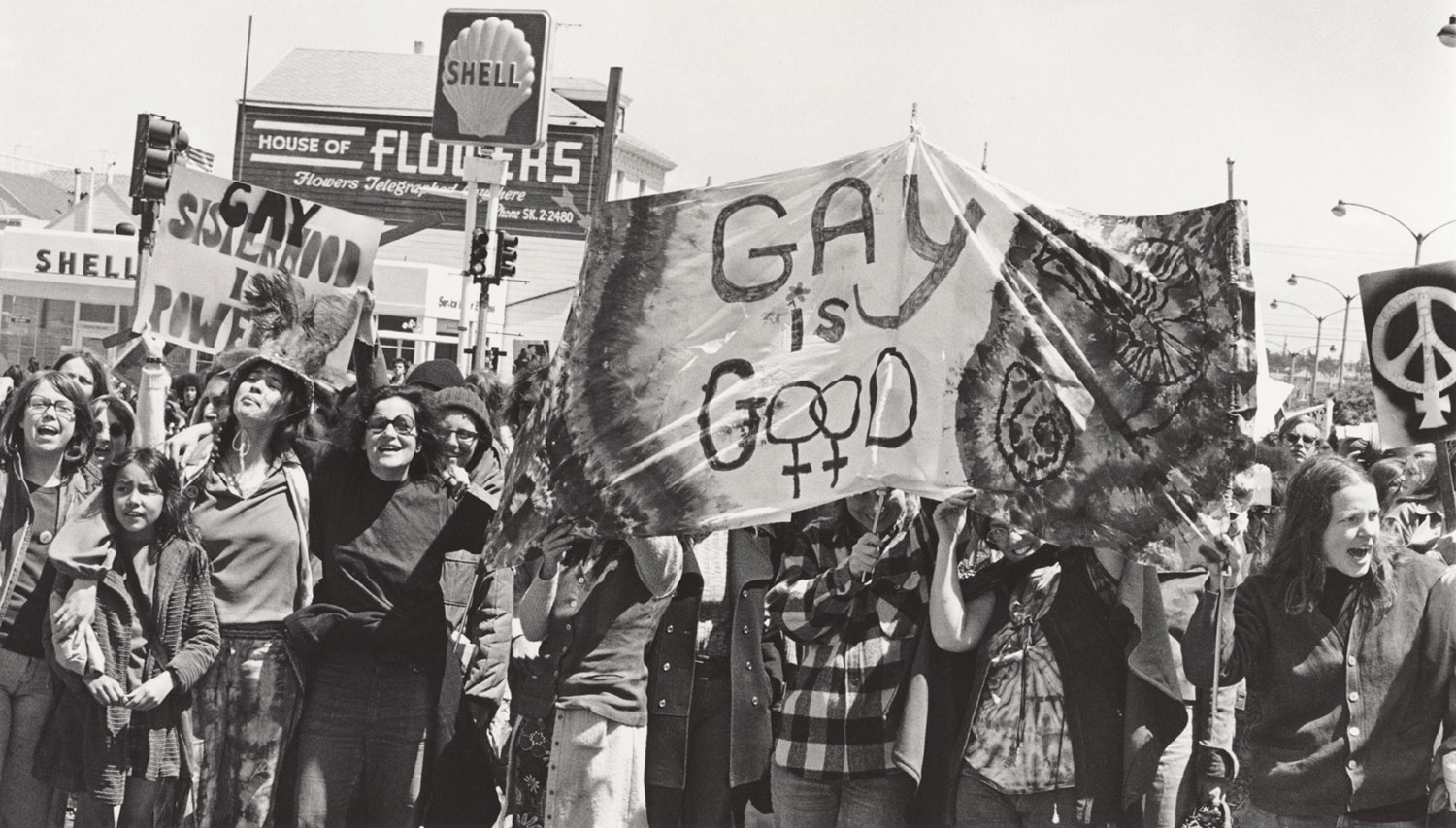This black-and-white photograph, likely taken during the 1970s, captures an evocative scene of a protest advocating for LGBTQ+ rights. Central to the image is a group of demonstrators, predominantly women with long hair, holding a large, tie-dye-inspired banner reading "Gay is Good," the O's stylized with astrological symbols resembling the Venus symbol. To the left, another prominent sign declares "Gay Sisterhood is Powerful." On the right side of the image, a distinct peace symbol can be seen, underscoring the era’s broader social movements. The backdrop features various advertisements, including a clearly visible Shell gas station sign and a building marked "House of Flowers," providing a poignant juxtaposition of everyday commerce with the urgent call for equality and acceptance.